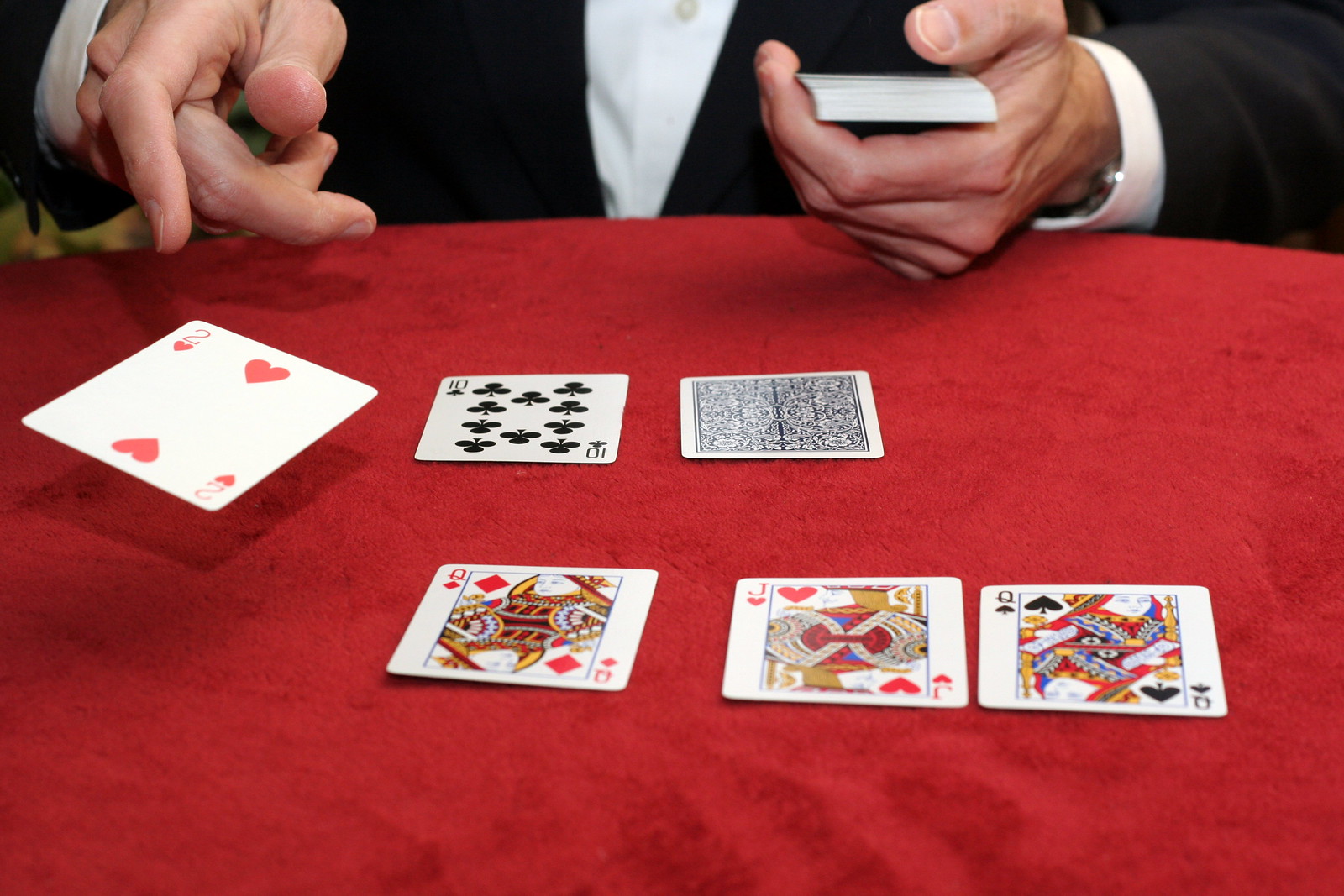The photograph captures an intense moment during a card game, taken from the perspective of someone seated across a circular table draped with a red cloth. At the top edge of the image, a man dressed in a black jacket over a white shirt is visible, his gaze focused on the cards in his hands. He is in the midst of dealing, with one hand gripping a deck of cards while the other has just flicked the Two of Hearts onto the table. Also visible on the tabletop are the Queen of Diamonds, the Jack of Hearts, the Queen of Spades, and the Ten of Clubs. An additional card lies face down, yet to be revealed. The cards are standard playing cards, featuring the classic depictions of the face cards and numerals. They appear new, each card vibrant and crisp, setting the stage for a high-stakes play yet to unfold.